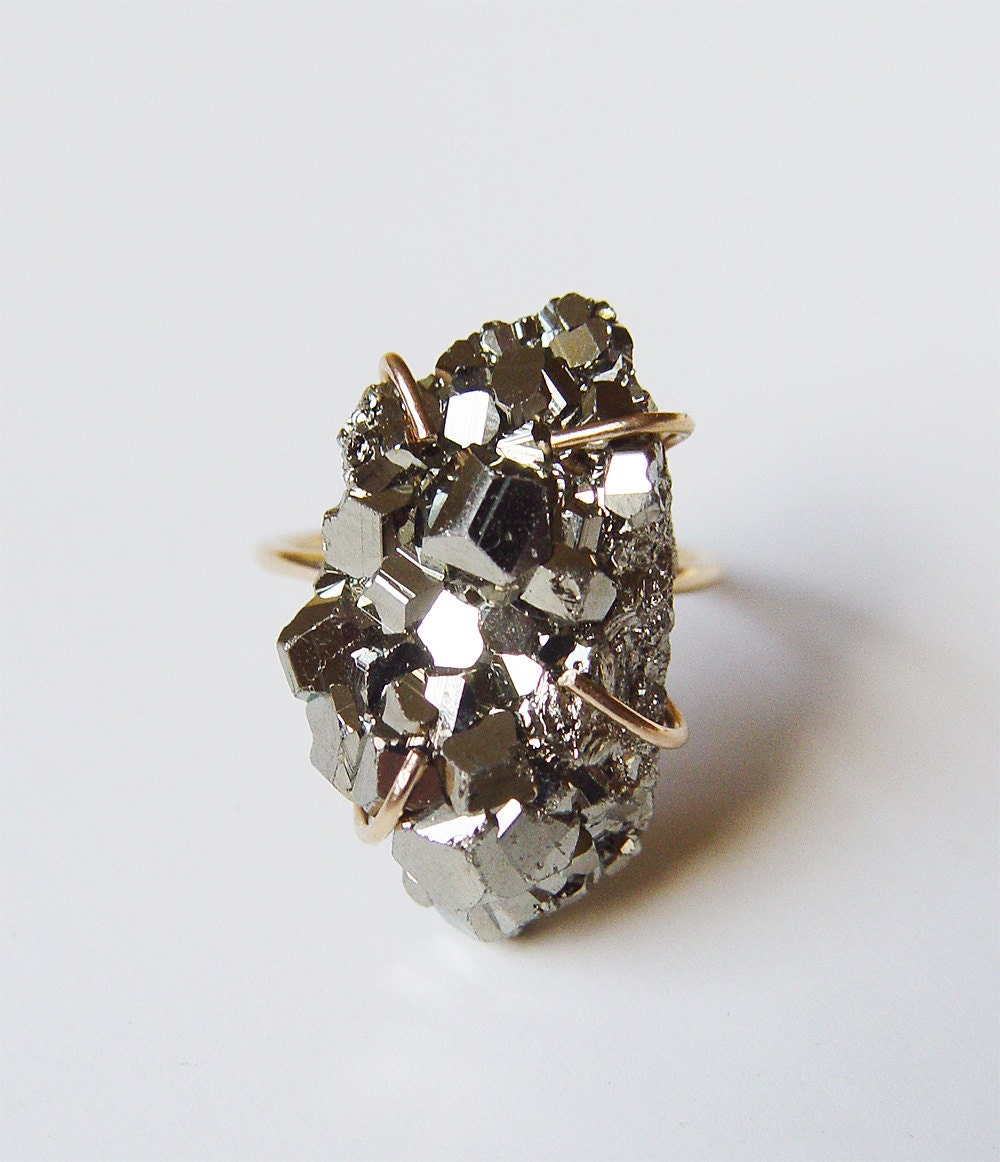The image showcases a high couture ring prominently displayed against a clean white background that appears slightly light gray due to the lighting. The ring features an intricate design with a large, raw, and natural dark gray metallic crystal as its centerpiece. This striking gemstone is encrusted with various shapes of smaller minerals and has a glistening, bumpy texture with numerous multi-faceted crystalline formations. The crystal, almost oval in shape and oriented vertically, is held securely by four elegant, gold claw-shaped prongs. Behind the sizable crystal, a slim gold band is partially visible but out of focus, adding to the prominence of the gemstone. The entire composition emphasizes the raw and irregular beauty of the metallic stone, making the ring appear as a luxurious and unique piece of jewelry. No text is present in the image, ensuring that all attention is on the detailed craftsmanship and the stunning mineral at the center.